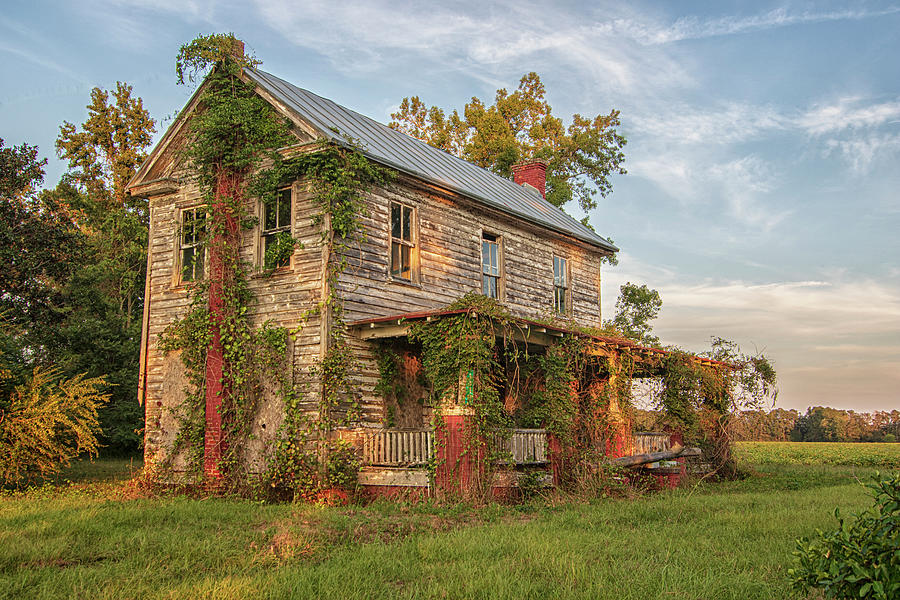The image depicts a dilapidated, two-story farmhouse set amidst overgrown grass and surrounded by deciduous trees. The wooden siding of the house is weathered, discolored to a faded gray and brown, and stripped of paint, lending it a deserted and abandoned look. The farmhouse features two distinct chimneys: a prominent red brick chimney overgrown with deep green and light green vines, and a smaller, gray sheet metal chimney visible at the crest of the roof on the right. The metal roof, dull and worn, tops the structure, which is built upon a brick foundation. 

A sprawling front porch, upheld by red brick pillars partially concealed by the overhanging roof, extends across the farmhouse. Wooden railings line the porch, which is also entangled with creeping ivy. The house has a total of five windows: three above the porch and two on the left side. The four-pane windows appear to be sliding types, with noticeable gaps in the upstairs panes, hinting at the house's state of neglect. 

In the foreground, the lawn is unkempt with high grass, while bushes flank the bottom corners—one to the right and one closer to the left side of the house. Behind the farmhouse, a dense line of deciduous trees, mostly green with some yellow-tipped foliage, frames the scene, and a mowed field stretches into the distance with additional trees lining its perimeter.

The sky above is a mix of cyan blue with white clouds dispersed throughout—larger clouds hover over the distant forest, and smaller streaks spread closer to the farmhouse. The weaker sun, casting long shadows across the landscape, suggests that the image is captured in the mid-afternoon or close to evening, contributing to the overall tranquil yet desolate atmosphere.